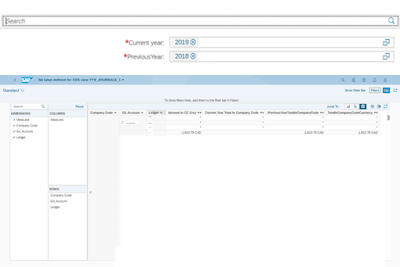The image primarily displays a user interface with several elements, though some portions are blurry and difficult to decipher. 

At the top is a search box highlighted with an icon of a magnifying glass, bearing the placeholder text "Search." Directly beneath this is a red asterisk followed by the label "Current Year," accompanied by an input box displaying "2019." Below it, another red asterisk marks the label "Previous Year" next to an input box displaying "2018."

Further down, there's a window distinguished by a light blue border along the top, containing the text "SAP" (though slightly unclear) with additional text alongside it. Beneath this window is a dropdown menu followed by another search box.

The layout includes three additional boxes below these elements: 

1. The leftmost box with four distinct entries.
2. The top-right box containing a single entry.
3. The bottom-right box listing three entries.

Along the right side of the interface are seven columns, the contents of which are indistinct.